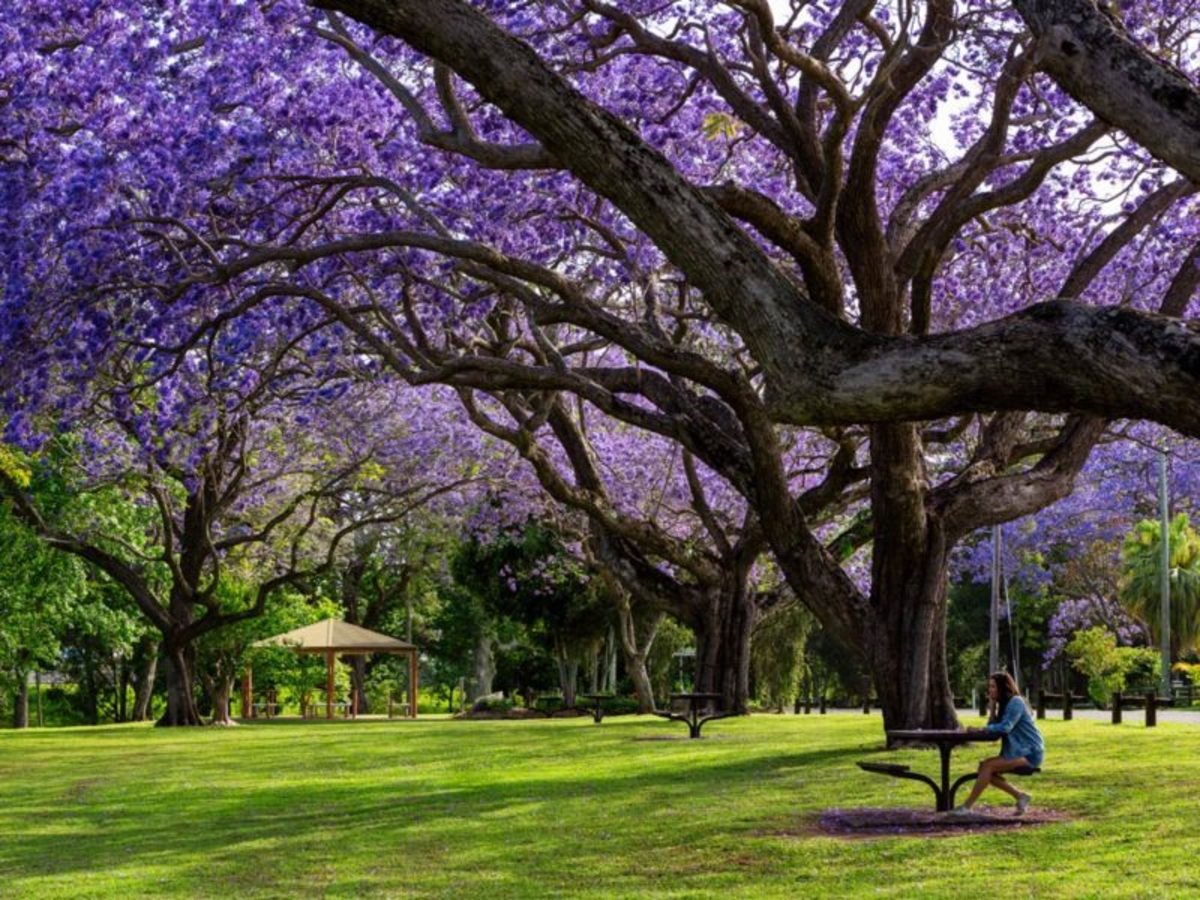In the outdoor park, the photo captures a serene scene beneath a canopy of flourishing jacaranda trees with their striking purple blooms dominating the upper portion of the horizontal rectangular image. Three prominent tree trunks emerge from the middle right and upper right, their thick branches reaching out, intermingling with the vibrant purple leaves. The ground is a lush, bright green grass that covers the bottom third of the image, intersected by shadows cast by the trees.

On the lower right, a woman with long brown hair is seated at a picnic table. She is wearing a blue long-sleeve top and white tennis shoes, and her hand is thoughtfully resting on her chin. Her knees are bent, suggesting she might be sitting on a bench. Behind her, there's another picnic table in the distance that remains unoccupied, adding to the tranquil atmosphere of the scene.

To the lower left of the picture, there is a covered area with additional picnic tables and a wooden gazebo further off, indicating the setting to be a large public garden or park. The scene is framed by trees, some of which have green leaves, creating a beautiful contrast with the dominating jacaranda blooms. The sky peeks through the upper right-hand corner, completing the peaceful, likely spring day captured in this image.